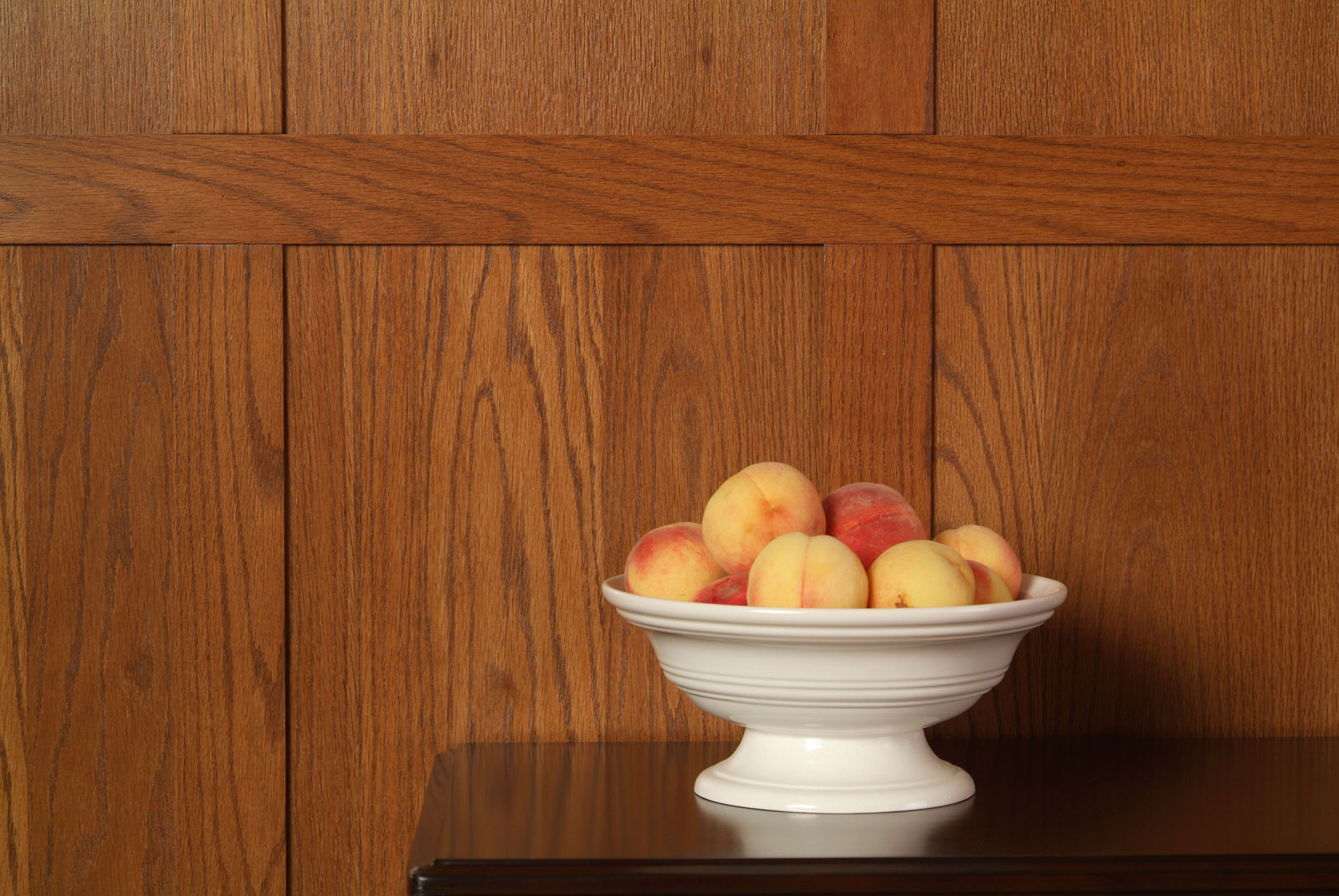In the image, there is a white porcelain or pottery bowl filled with eight peaches, which display shades of yellow, light peach, and some hints of red and orange. The bowl is positioned toward the middle right side of a highly polished, black wooden table, showcasing a mirror-like finish. This table is part of an indoor setting, likely a living room, and is placed against a dark, wooden, paneled wall that features visible grain, two vertical panels, and a horizontal trim. The overall scene captures a rustic yet polished aesthetic, highlighting the contrast between the rich wood textures and the vibrant, fresh peaches.